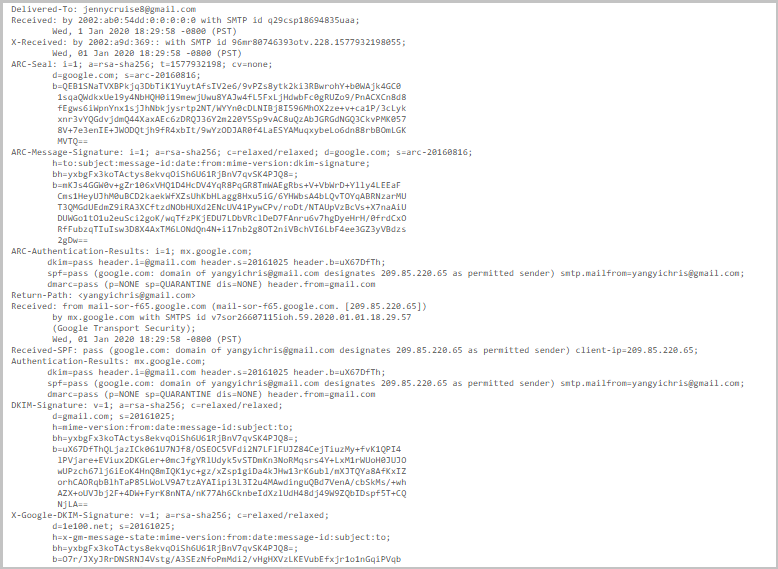The image showcases an email header displayed against a plain white background. The content consists of numerous intricate technical details typically found in email metadata. The email appears to be delivered to jennycruze@gmail.com and received by the domain 2002 ABC. There is a prominent blue outline framing the entire image, with the blue border being more intense on the left and top edges, and gradually fading on the right and bottom edges. The email header includes various fields such as recipient and sender information, numerous numerical and alphanumeric codes, and multiple authentication details. Among the key elements listed are "return-path," "received-SPF," "DKIM signatures," "X-Google," and "authentication results." Overall, the image is dense with technical jargon, all meticulously presented within the outlined blue border.